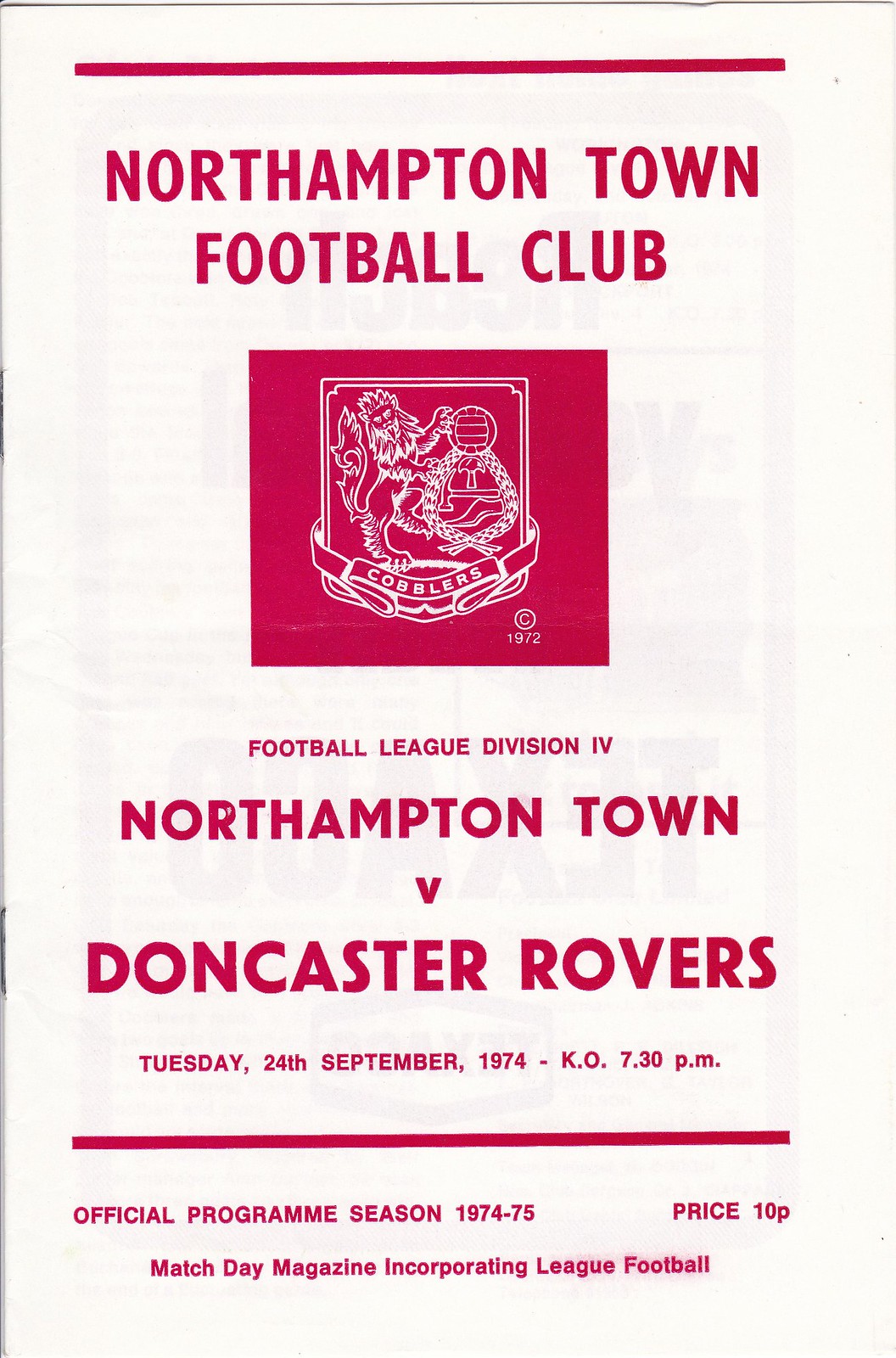This vertical rectangular image features the cover of an official program for a soccer match, sporting a clean, white background with dark pink or light red text and lines. At the top, a red line frames the text "Northampton Town Football Club" in large letters, indicating the poster's focus. Directly beneath this title is a red square containing the Northampton Town Football Club's coat of arms, prominently centered slightly above the middle of the image. The crest features a banner inscribed with the word "Cobblers."

Below the coat of arms, in smaller print, "Football League Division 4" is indicated, followed by the announcement of the match: "Northampton Town vs. Doncaster Rovers." The event is scheduled for Tuesday, 24 November, 1974, with a kickoff time of 7:30 PM. Additional details at the bottom of the poster outline that this is the official program for the 1974-75 season, priced at 10p, and part of a match day magazine incorporating league football. Another red line marks the division between this main information and further smaller print below.